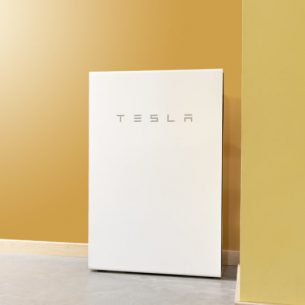This pristine image showcases a sophisticated setting dominated by a minimalistic, high-end aesthetic. Central to the composition is a white plaque or sign positioned against a golden yellow wall with a neat white baseboard. The plaque itself features the iconic "Tesla" name, elegantly rendered in sleek gray letters, symbolizing the brand’s reputation for innovation and luxury. The surrounding floor is a contrasting gray, adding to the modern and exclusive ambiance of the scene. The bright lighting in the room accentuates the clarity and premium feel of the environment, reflecting Tesla's prestigious and elite status.